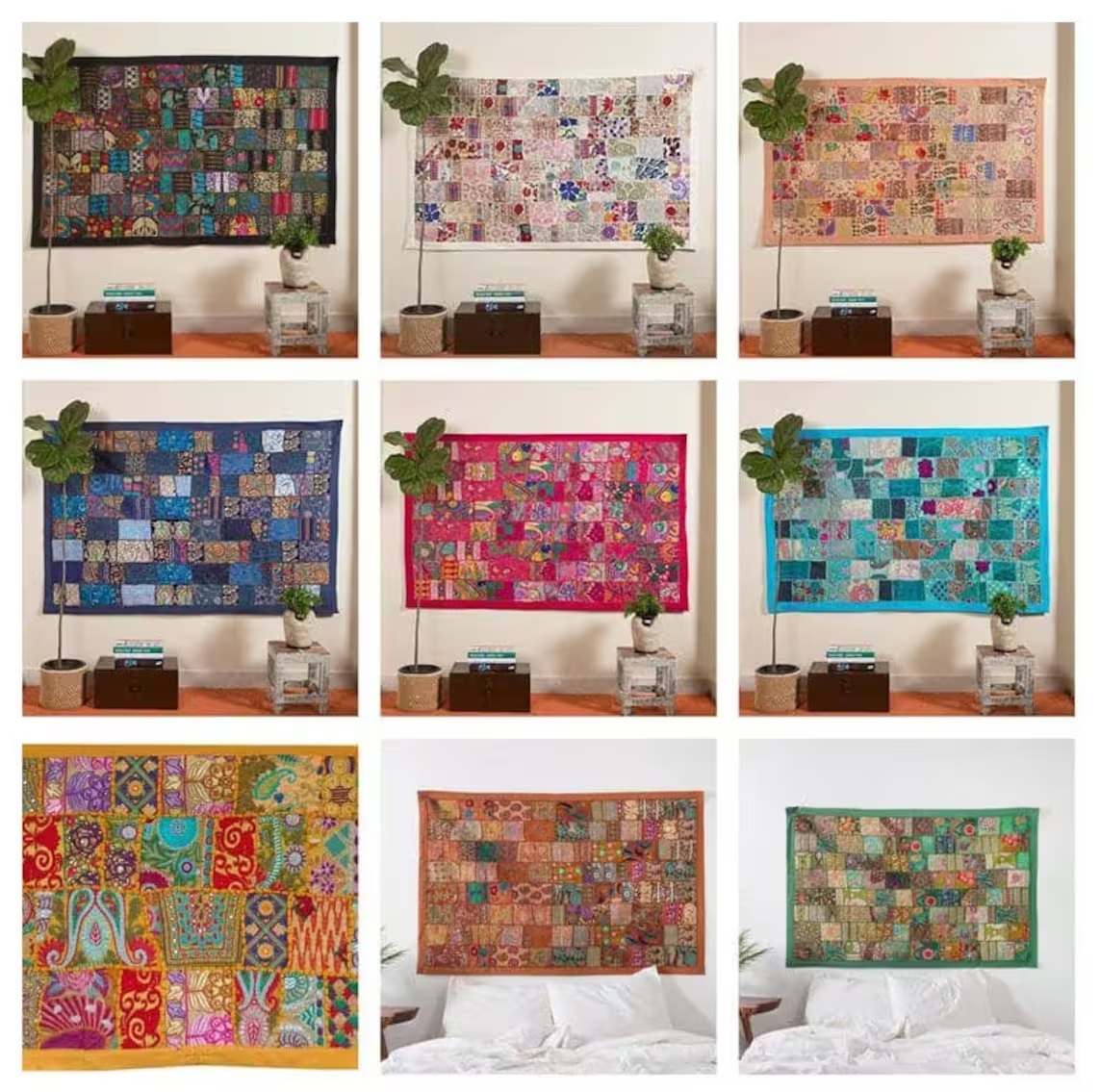This image collage features nine individual photos arranged in three horizontal rows of three, each showcasing a unique quilt. In the top two rows, each quilt is displayed hanging on a light or tan wall. A tall potted plant with a narrow trunk and large green leaves is positioned on the left side of these six images, accompanied by a table on the right. The table holds a smaller potted plant in a white clay vase. The quilts in these rows exhibit a variety of colors and patterns including dark pinks, blues, whites, and browns.

The bottom row consists of three images: the first one on the left shows a full-view quilt with no other elements in the frame. The other two images depict quilts draped behind a bed with white bedding and pillows, allowing only the edge of a side table and plant to be visible. The quilts above the bed contrast in color, one being brownish-tan and the other green. This collection of images highlights the diverse designs and settings of each quilt in a well-lit, minimalistic room.